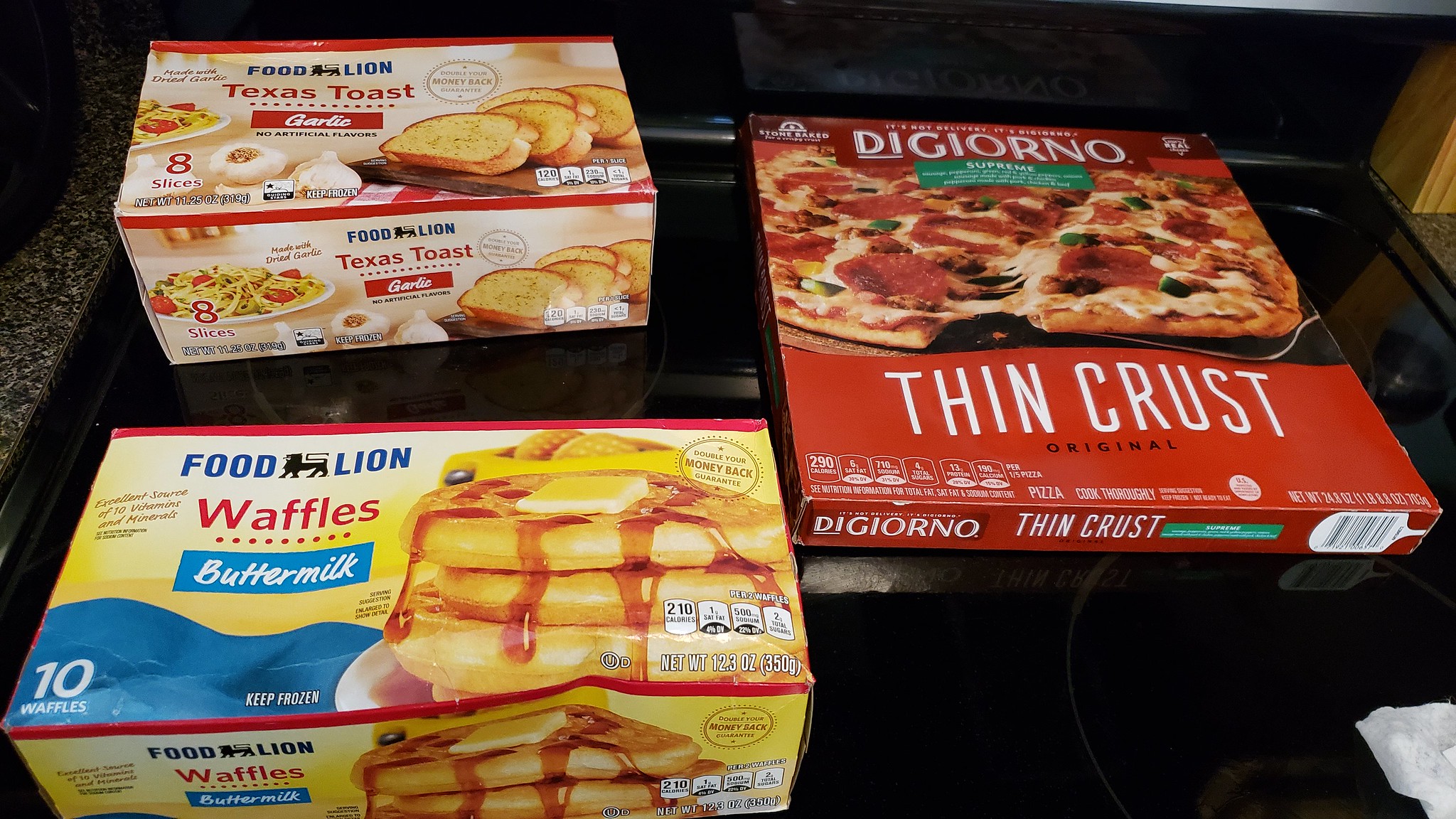In this photograph, three distinct boxes of frozen foods are displayed on a sleek, black, and reflective stovetop, with the surrounding edges revealing a polished granite countertop. In the lower left corner, a box of Food Lion frozen waffles is prominently featured. The front of the box showcases an appetizing image of a stack of golden waffles generously topped with melting butter and syrup, along with the Food Lion logo and a product description. 

In the back left corner, a box of garlic Texas toast stands out. The packaging is adorned with enticing visuals, including slices of crispy garlic bread, a serving of pasta, and fresh garlic bulbs, hinting at the rich flavors inside. 

On the right side of the stovetop, a vibrant red-colored box containing a DiGiorno thin crust pizza captures attention. The box presents a meticulously styled image of the pizza, emphasizing the thin, crunchy crust and an abundance of savory toppings. 

The overall composition of the photograph highlights the variety of frozen meal options available, skillfully arranged against the modern kitchen backdrop.